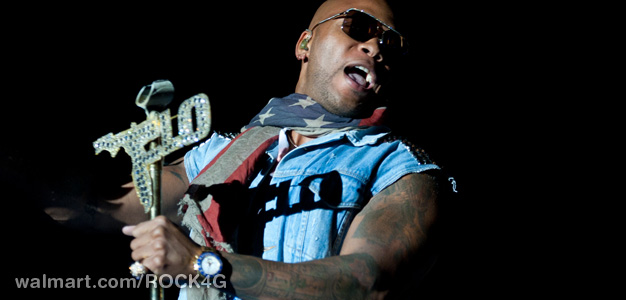This detailed photograph captures a bald man, seemingly in his 40s or 50s, performing on stage against a black background. He wears dark-tinted glasses and a sleeveless blue denim shirt with the sleeves torn off, complemented by an American flag scarf around his neck, which intriguingly features gray, blue, and red colors instead of the traditional red, white, and blue. His tattooed arms are visible, and his left hand, adorned with a white-centered blue-rimmed watch, grasps a silver microphone stand. The microphone itself displays a rhinestone logo spelling "FLO," with the 'F' shaped like the state of Florida, hinting at a possible reference to Flo Rida. The man's mouth is open, suggesting he is either singing or speaking, and he is leaning back slightly, looking to the side. In the bottom left corner, the watermark "walmart.com/rock4g" is semi-transparently imposed over the image.